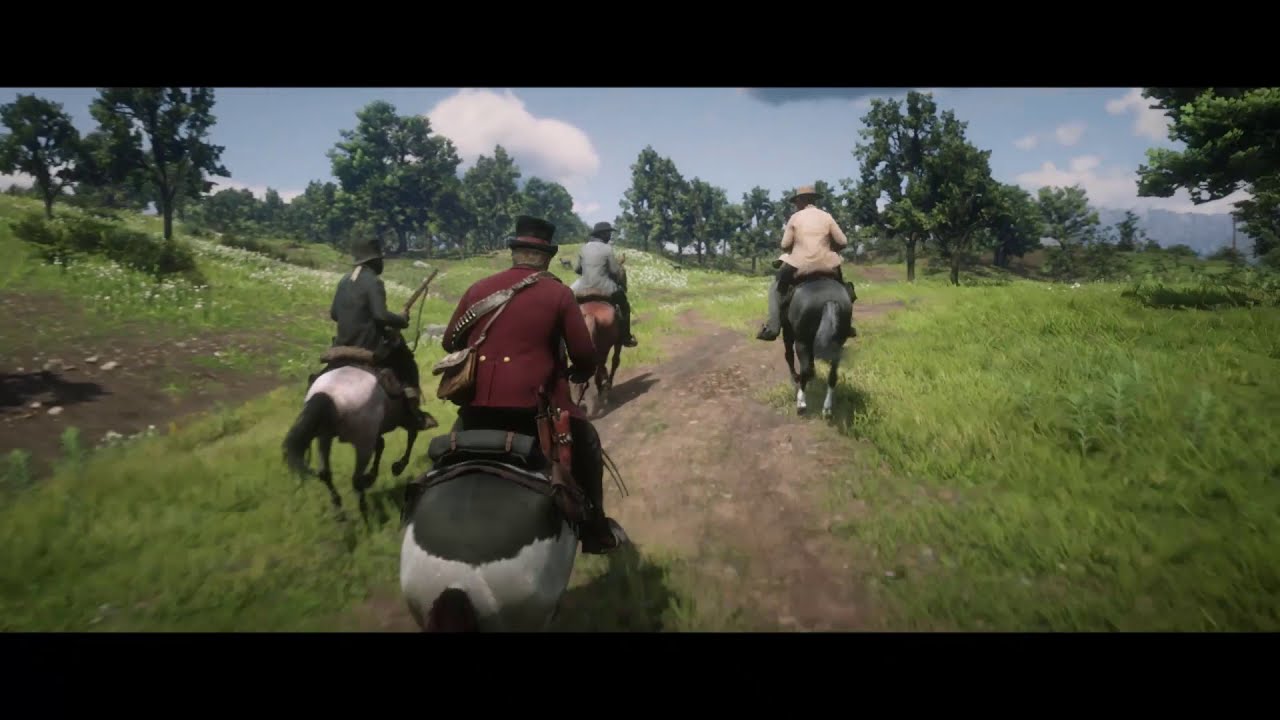The image is a screenshot from what appears to be the video game Red Dead Redemption, depicting a western setting. Four horsemen are riding away from the camera along a dirt path through a meadow dotted with scattered trees. The sky is blue with fluffy white clouds. The closest rider is centrally positioned, wearing a burgundy suit with red buttons and a black top hat, and is mounted on a black and white horse. To his left is another rider dressed in dark clothing and a black hat, holding a shotgun and riding a white horse. In front of them, a rider on the left is in a gray jacket with a dark hat, on a grayish horse, while the rider on the right wears a tan jacket and hat, and rides a gray horse. The scene is bordered by black strips at the top and bottom of the image.